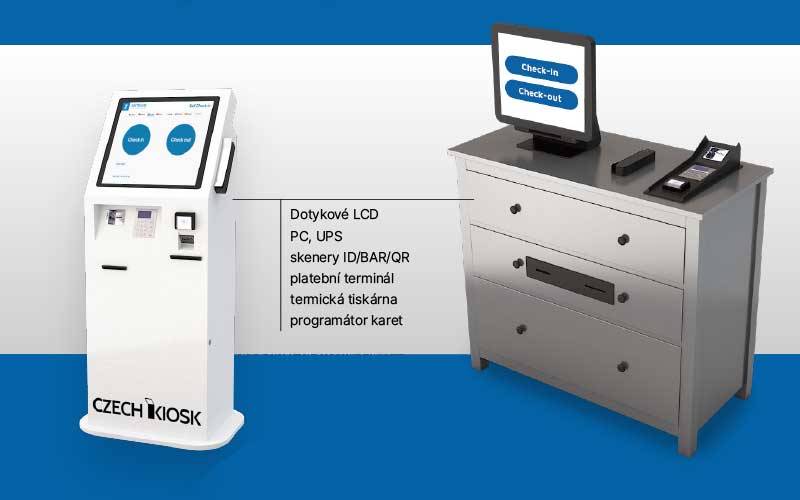This image appears to be a detailed infographic set inside a business environment, featuring various elements on a blue floor with a dual-band blue and white background. Dominating the left side of the image is a sleek white kiosk labeled "CZECH KIOSK" at its base. This kiosk has a touch screen bordered in black, displaying two large blue circles with the labels "Czech In" and "Czech Out" in white font. 

In the center of the image, black text written in what appears to be the Czech language provides information, including terms "LCD" and "PC" in English. An arrow from this text points to the right side, connecting to a gray three-drawer cabinet angled slightly to display both its front and side. Atop this cabinet is a black-bordered monitor showing a white screen with two blue, rounded rectangles carrying the labels "Check In" and "Check Out" in white, matching the color of the floor.

The cabinet also supports two additional office items, one being a black rectangle likely a card scanner, and another black-and-white object that resembles a stapler. The overall style and layout of this image suggest it is a presentation slide, comparable to something one might see in a PowerPoint presentation, likely illustrating the setup and function of a check-in/check-out system.